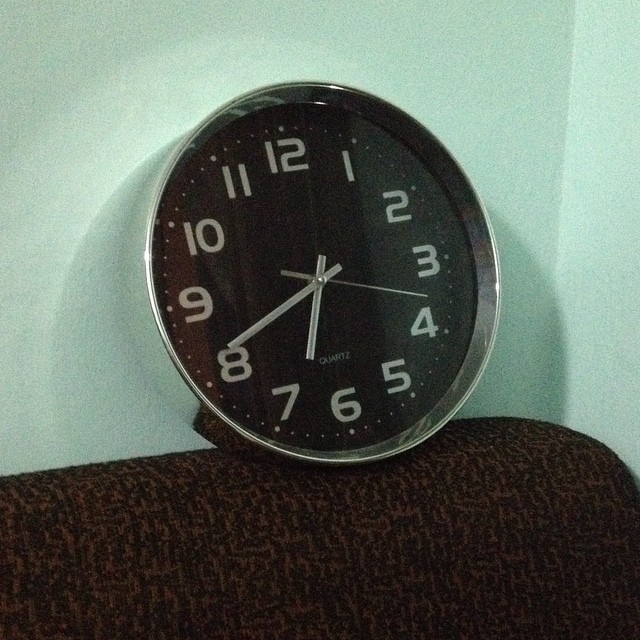This detailed colour photograph, taken indoors under poor lighting conditions, appears quite grainy and may have a filter applied, giving the scene a desaturated, almost colourised black-and-white look with prominent green, brown, and black hues. At the center of the image is a round clock, perched precariously on the back edge of a curved brown chair or couch with a dark brown print and black edging. The clock sits against a pale green wall, which casts shadows on either side. The clock face features light-colored numbers from 1 to 12 with a greyish-greenish tint and slivery grey hands pointing to 6:40. A smaller second hand is positioned between the 3 and 4 o'clock marks. The clock's rim is silver metallic, reflecting small sparkles of light. Below the clock, a small stand supports it against the wall, rather than it being mounted directly.